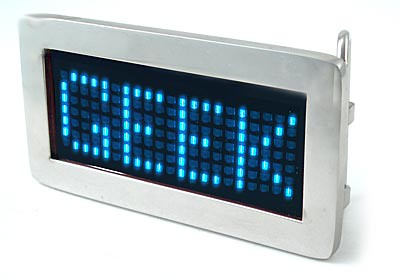This image features a sleek, metallic rectangle with a polished silver finish. The perspective of the photo showcases the flat face of the rectangle, with a slight tilt making the left side appear to recede behind the right. Dominating the center is a prominent black rectangle, which serves as a backdrop for the word "GEEK," spelled out in vibrant blue digital letters. The letters are composed of individual illuminated squares, each glowing a light blue hue. To the right of this central feature are two smaller silver squares, positioned one near the top and another near the bottom, adding a touch of symmetry and balance. Along the right edge of the rectangle runs a slender silver cylinder, extending slightly beyond the upper right corner, curving gently upwards before disappearing behind the top edge. The meticulous design and arrangement of these elements suggest a high-tech device or an artistic representation of digital technology.